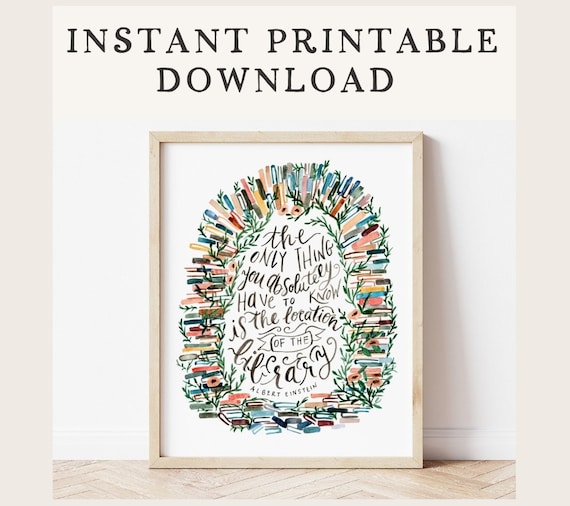This photograph captures a framed piece of art propped against a white wall, resting on a light beige wooden surface that appears to be either a table or floor. The artwork is encased in a simple, narrow wooden frame matching the surface below. At the top of the image, the words “Instant Printable Download” are prominently displayed. The artwork itself features an oval shape comprised of vertically and horizontally placed books, arranged in a manner that resembles leaves or multicolored bars radiating from the center. The center is white and bears a quote in elegant, loose cursive script that reads, “The only thing you absolutely have to know is the location of the library,” attributed to Albert Einstein. This piece would appeal to book lovers and can be saved on a computer for printing, offering both a visually pleasing and inspiring message.